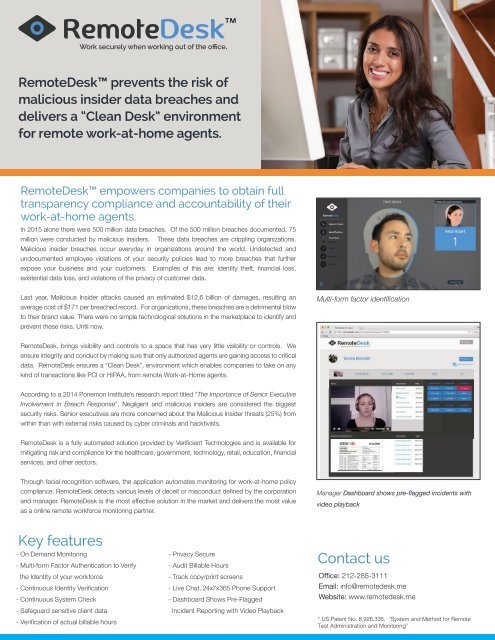This advertisement promotes "Remote Desk," highlighting its ability to enhance security and compliance for remote work environments. The logo features a diamond with a blue circle, with the words "Remote Desk" in navy blue and light blue, and the trademark symbol. The tagline emphasizes secure remote office work, stating: "Work securely when working out of the office."

Remote Desk addresses the increasing risk of data breaches, particularly from malicious insiders, which caused significant damages in recent years. In 2015, out of 500 million data breaches, 75 million were conducted by malicious insiders, resulting in an estimated $12.6 billion (with a 'B') in damages last year, and an average cost of $171 per breached record.

A 2014 study by the Ponemon Institute, titled "The Importance of Senior Executive Achievement in Breach Response," underscores that negligent and malicious insiders are the biggest security threat, with senior executives being more concerned about internal risks than external cybercriminals.

Remote Desk employs facial recognition software and automated monitoring to ensure compliance with work-at-home policies, detecting various levels of deceit and misconduct as defined by the corporation and managers. It's touted as the most effective solution on the market for remote workforce monitoring.

Key features of Remote Desk include: on-demand monitoring, multi-form factor authentication to verify workforce identity, continuous identity verification and system checks, safeguarding sensitive data, verifying actual billable hours, privacy security, auto-eligible hours tracking, copyright screen tracking, live chat support 24/7/365, phone support, and a manager dashboard that shows pre-flagged incidents with video playback.

The advertisement features images of people working remotely: a man, a woman with headphones, and an attractive woman smiling while leaning on a desk. For more information, viewers are encouraged to contact the company via their office number, email, or website.